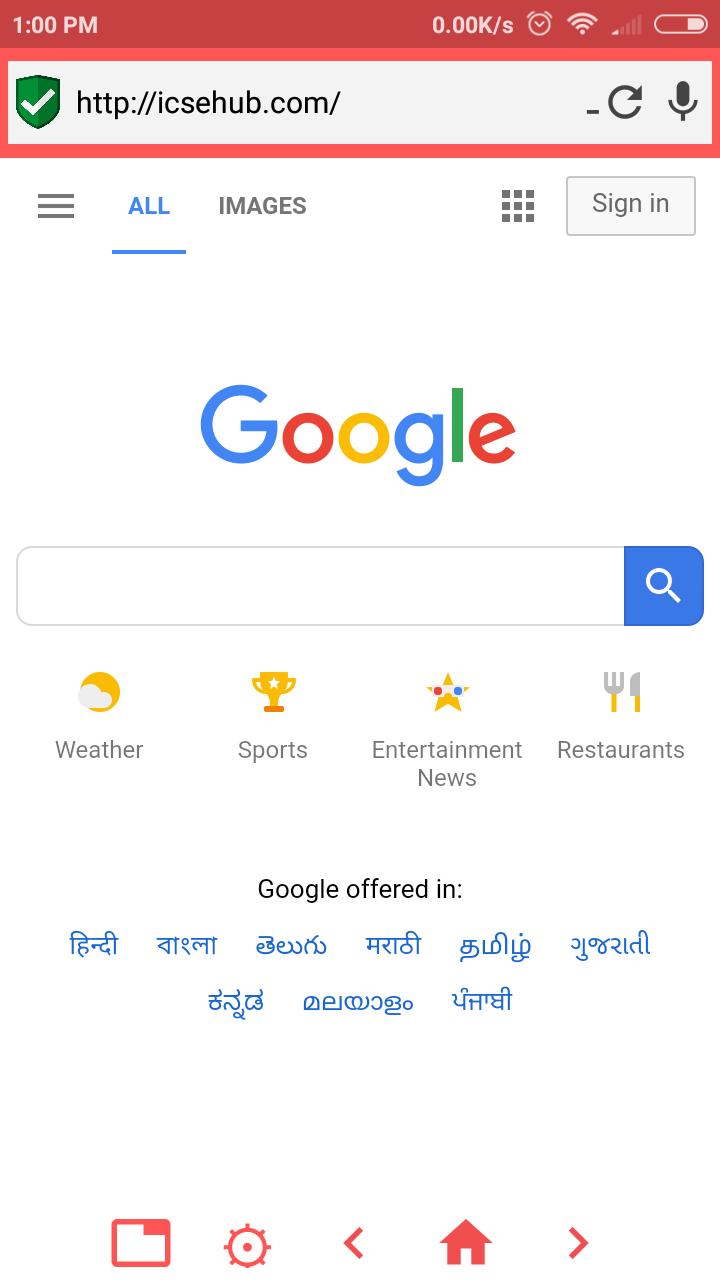Screenshot of Google Home Page at 1 PM

This detailed image shows a smartphone screenshot of the Google home page captured at 1 PM. At the top of the screen, there's a red status bar displaying a clock icon, Wi-Fi signal icon, and a battery icon. Below the red banner, there's a Google search bar featuring a green security check shield and a microphone icon. To the left of the search bar, there's a 'hamburger' menu icon, followed by the 'All' tab in the center, indicating the active tab, and the 'Images' tab next to it.

Directly below the search bar, there are several boxes representing other apps within the Google ecosystem, and next to them is a 'Sign in' button. Moving further down, the colorful Google logo is prominently displayed. Beneath the logo, there is another search bar ready for user input.

Underneath the search bar, the interface displays quick access icons: a weather icon with a forecast, a trophy icon labeled 'Sports', a star icon for 'Entertainment News', and a fork and knife icon tagged 'Restaurants'.

Towards the bottom of the screen, black text reads, “Google offered in” followed by text in another language indicating additional language options—though the specific language is not identified.

Finally, at the very bottom of the screen, there is a navigation bar with icons including a screen icon, a settings gear icon, a left-facing arrow, a home icon, and a right-facing arrow, all colored in red.